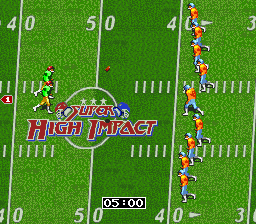In this still image taken from an American football video game, players are seen competing on a vibrant green grass or turf football field. Painted yard lines marking the 30, 40, and 50-yard points are clearly visible, adding a touch of authenticity to the scene. A black bar at the bottom of the screen indicates that there are five minutes remaining in the game. The teams are distinguishable by their uniforms: one team is wearing green jerseys with red helmets, while the opposing team sports orange jerseys and blue helmets. The focal point of the image is a football, suspended mid-air, suggesting it has either been thrown or kicked towards the center of the field, capturing an intense moment of play.